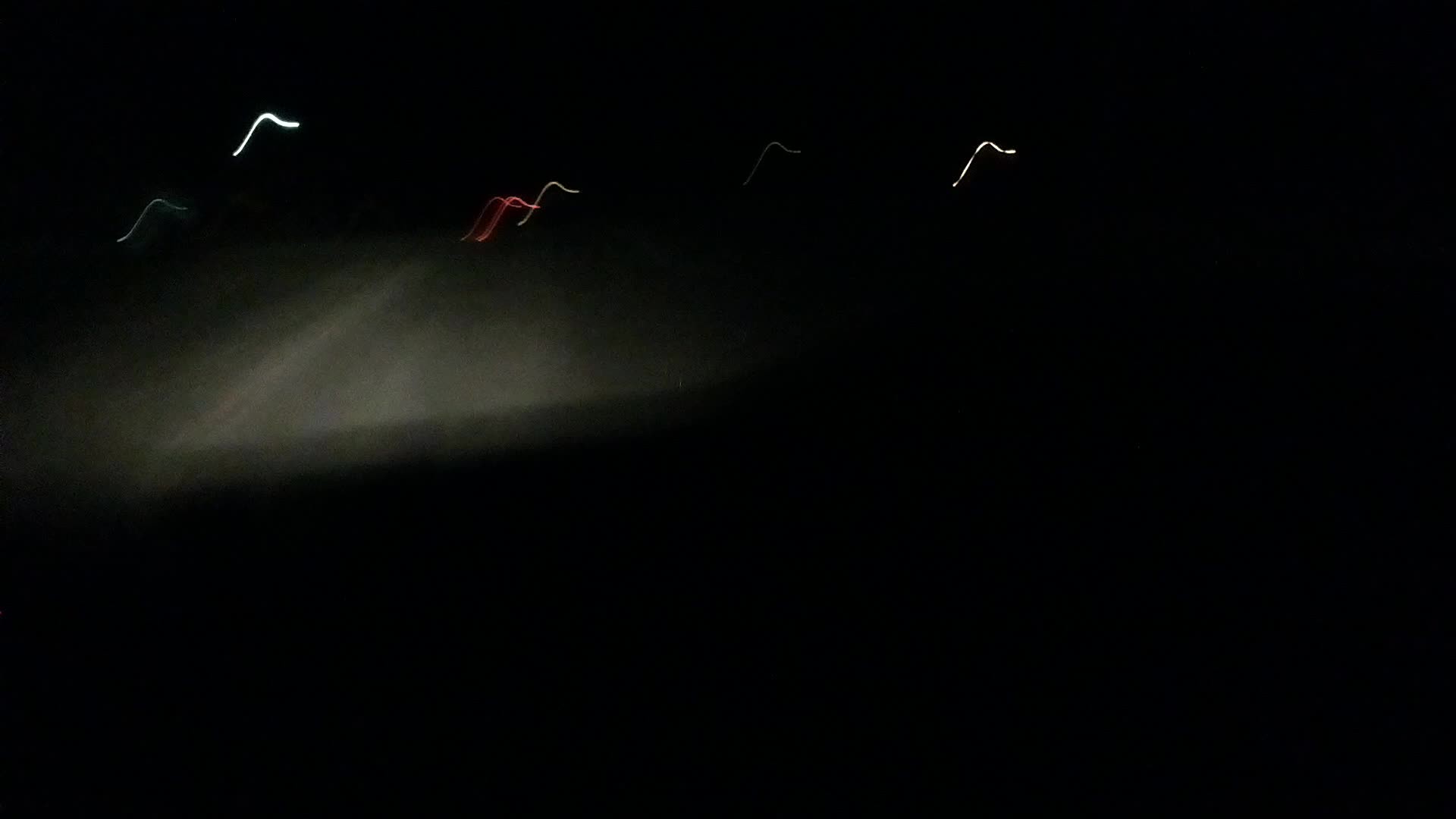A dim and blurry nighttime photo capturing the view from behind a car's windshield as it drives down a dimly lit road, the scene illuminated solely by the vehicle's headlights. The lower right portion of the image features a solid black area extending almost entirely across in a straight line, slightly angling down on the left side. In the upper left quadrant, a motion blur hints at the movement of the road. The top portion of the photo is punctuated by squiggles of bright lights, likely reflections from streetlights or passing vehicles, adding an abstract element to the scene.